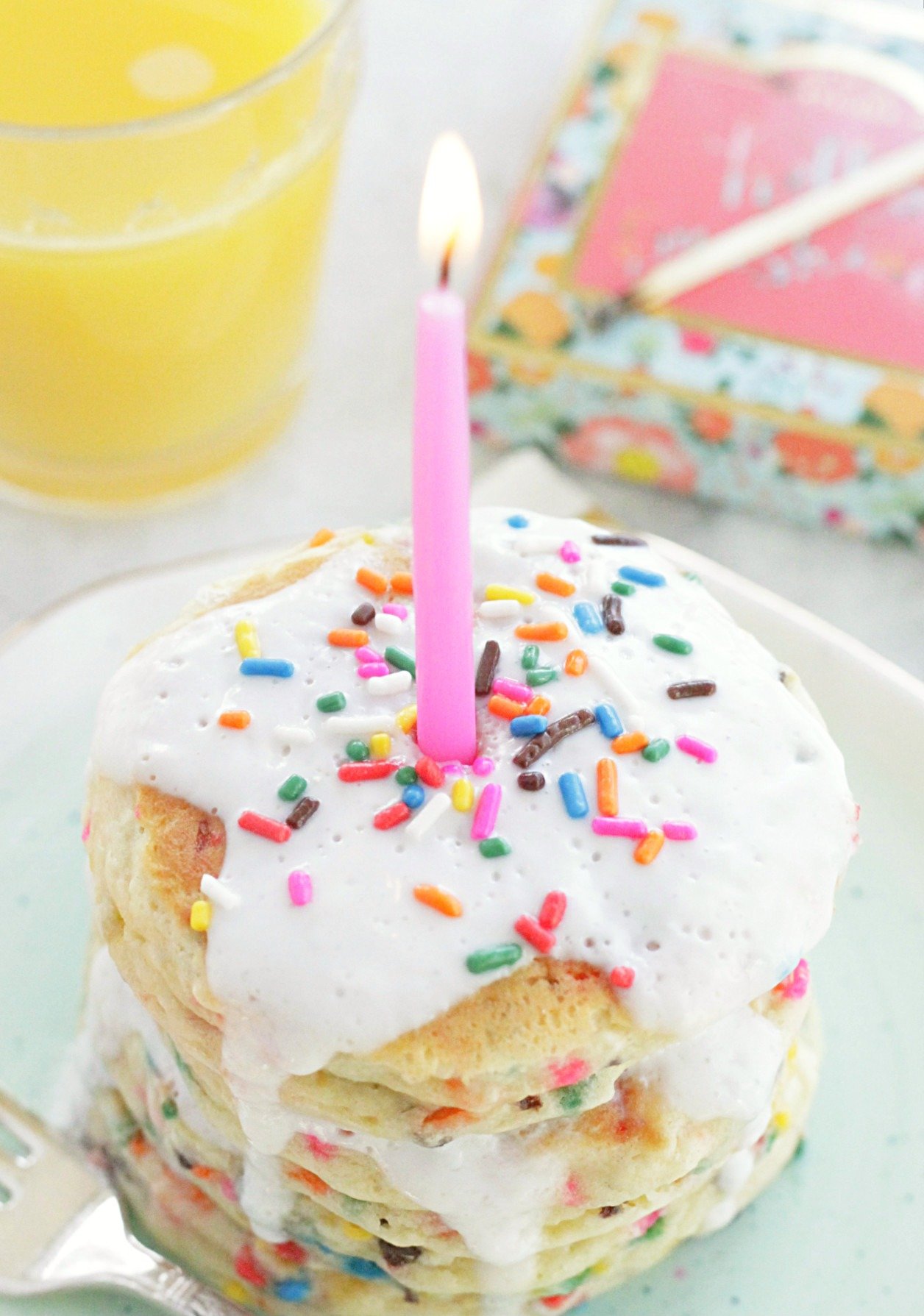A festive breakfast scene features a stack of approximately ten small pancakes arranged to resemble a birthday cake, topped with white icing and colorful sprinkles in hues of purple, red, brown, green, yellow, and blue. A lit pink candle sits proudly in the center of the stack. The pancakes, infused with rainbow confetti colors, rest on a white plate accompanied by a fork placed at the bottom left corner. To the top left of the image, a clear glass of what appears to be orange juice adds a refreshing touch. On the right side, a slightly blurred stack of birthday-themed napkins, possibly adorned with flowers, complements the celebratory setting. The image captures the bright and cheerful ambiance, though the focus is sharpest on the pancakes, with the background elements slightly blurred.